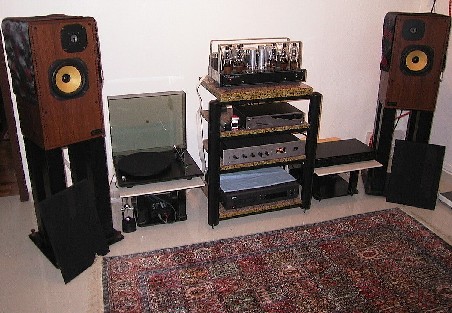This photograph captures a detailed view of a living room that serves as a dedicated music room. The centerpiece is a well-organized collection of stereo equipment positioned against a light cream-colored wall. Each side of the room features large stereo speakers with wooden sides; their covers are removed, revealing golden mid-range speakers and black tweeters. 

The stereo setup is showcased on a central rack that hosts various components: a turntable on a pedestal, a black component likely to be an equalizer or preamp, and possibly an old tape deck. A notable item on top of the rack is what appears to be a vintage tube amplifier, characterized by visible vacuum tubes.

The floor boasts a Persian rug with a mix of red and dark gray hues laid over brown-tan linoleum. Additionally, there's a chest positioned against the wall with multiple gold and silver items displayed on it. This equipment-filled room, devoid of people, effectively highlights its purpose as a space devoted to music, adorned with a mix of old and potentially modern audio technology.